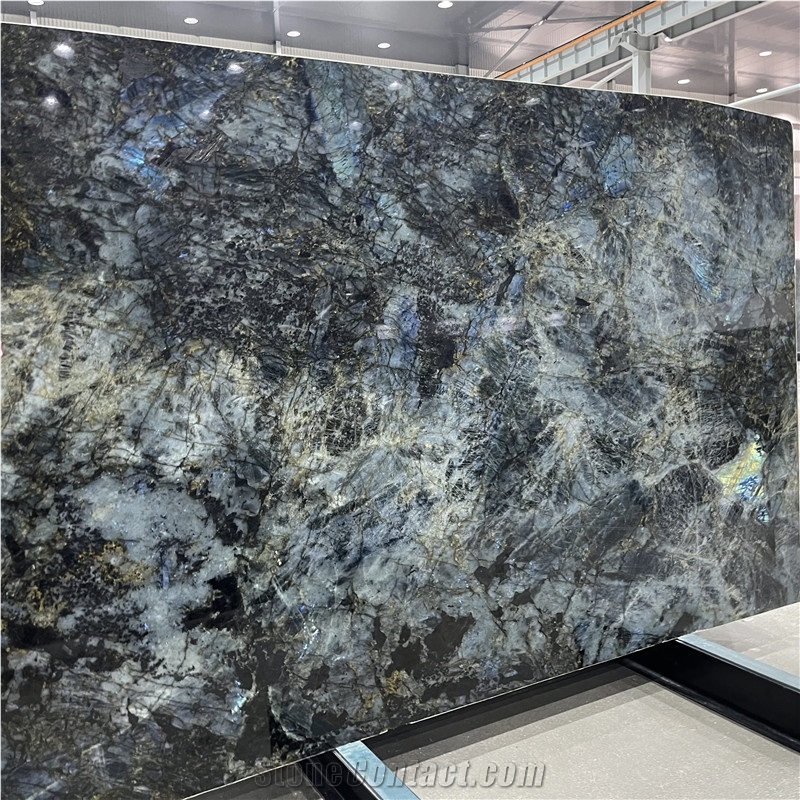The image depicts a large, horizontally-oriented slab that appears to be either a painting or a substantial piece of marble, resting on two metal bars laid on the ground for support. The slab takes up almost the entire frame of the image, showcasing an abstract and intricate pattern that combines dark blues, blacks, and light blue hues, with accents of yellow and gold. This detailed design could be reminiscent of a rocky or mountainous surface. The setting is a spacious room, likely a warehouse or a factory, evidenced by the high ceiling adorned with white beams and LED lights. Steel grey ceilings along with iron bars, pillars, and railings are visible in the background. At the bottom of the slab, there is a watermark reading "stonecontact.com," confirming that it is indeed a large piece of dark, patterned marble.